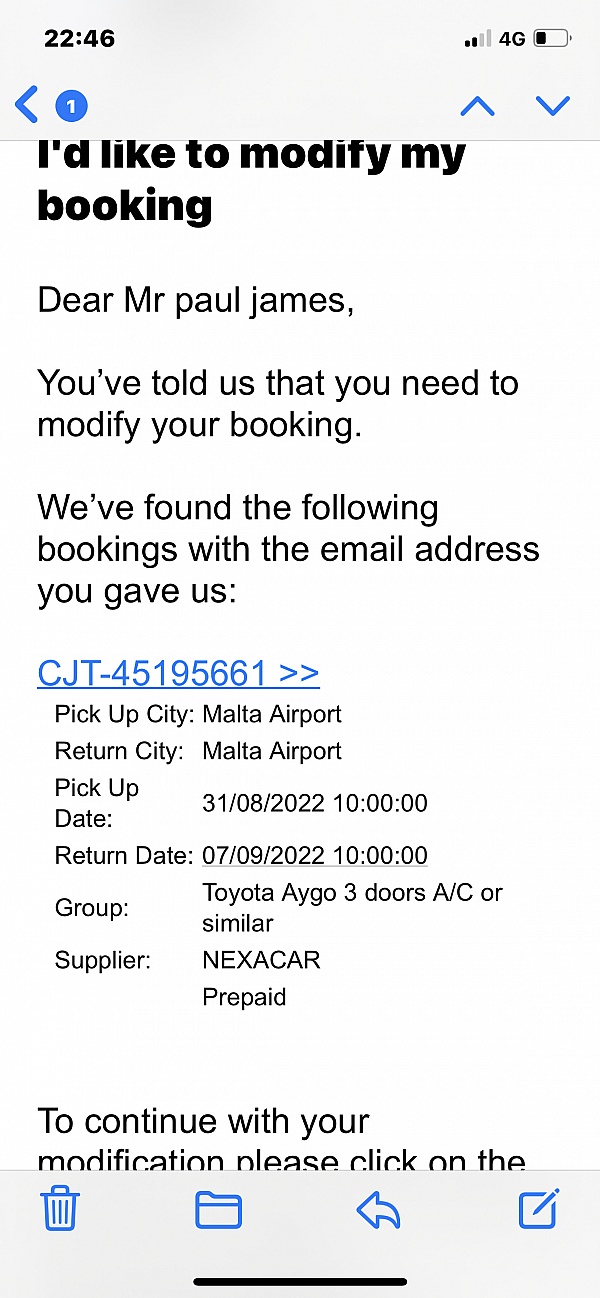The image captures a cell phone screen displaying a reply to an email or text message. 

At the top left corner of the screen, the time is indicated as 22:46. The top right corner features icons for cellular connection and battery status, which shows a nearly depleted battery and a "4G" network connection. Just below these, there's a small blue arrow pointing to the left and a number "1" inside a blue circle, indicating a notification.

The main body of the message is shown in large black text, starting with the statement, "I'd like to modify my booking." The message reads: "Dear Mr. Paul James, you've told us that you need to modify your booking. We've found the following bookings with the email address you gave us." The booking details are listed in blue text:
- Booking reference: CJT-451-95661
- Pick-up city: Malta Airport
- Return city: Malta Airport
- Pick-up date: 31-08-2022, 10:00
- Return date: 07-09-2022, 10:00
- Group: Toyota Ego three doors, AC or similar
- Supplier: Nexacar, prepaid

The message continues with an instruction: "To continue with your modification please click on the..." but the remaining text is obscured and not visible.

At the very bottom of the screen, the lighter gray background hosts four blue icons, aligned from left to right. These icons depict (from left to right):
1. A trash can
2. A folder
3. A left-pointing arrow
4. A square with a pencil going through it, indicating an edit option.